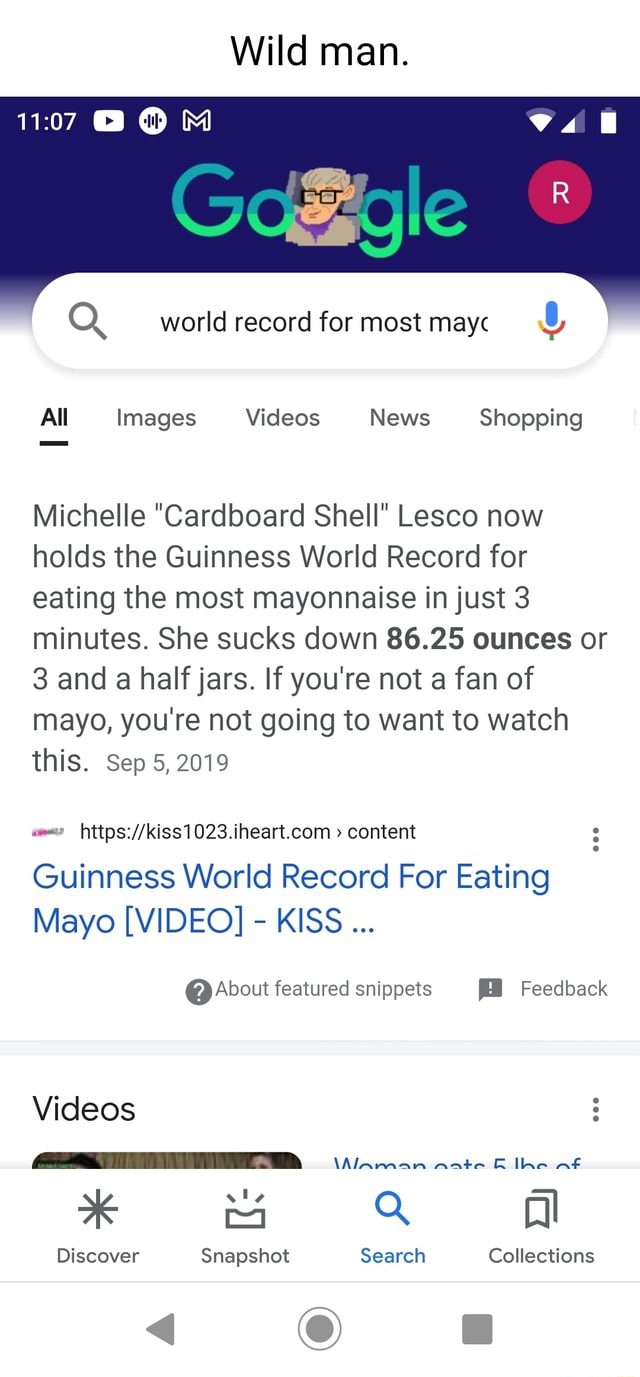**Detailed Caption:**

The screenshot showcases a smartphone screen featuring a Google search interface with an active video playback at the top. The phone's status bar at the top displays the time as 11:07 and shows connectivity icons indicating a two-bar Wi-Fi signal and a fully charged battery. 

The Google logo in this interface is a special Google Doodle comprised of a dark blue background with gradient lettering. The Doodle forms the word "Google" with unique representations: "G" followed by "O," a depiction of Stephen Hawking in place of the second "O," and "G-L-E" transitioning from dark to light green. Additionally, an "R," likely representing the Rakuten app icon, is also visible alongside the Doodle.

Beneath the Doodle, the search bar reads "world record for most mayonnaise," though it initially displays "world record for the most mayo." Below this, the search results headline reads: "Michelle 'Cardboard Shell' Lesco now holds the Guinness World Record for eating the most mayonnaise in just three minutes. She consumes eighty-six point two five ounces or three and a half jars. If you're not a fan of mayo, you're not going to want to watch this." 

Following this, there is a link to a Guinness World Record video titled "Dash Kiss" about eating mayo. The interface also includes various options like 'All,' 'Images,' 'Videos,' 'News,' and 'Shopping.' Additionally, there is a 'Featured Snippets' feedback section. Near the bottom, there is another video suggestion that mentions a woman eating five pounds of an unspecified item. Lastly, the bottom navigation bar of the interface features options for 'Discover,' 'Snapshot,' 'Search,' 'Collection,' 'Back,' and the play/currently active video control buttons.